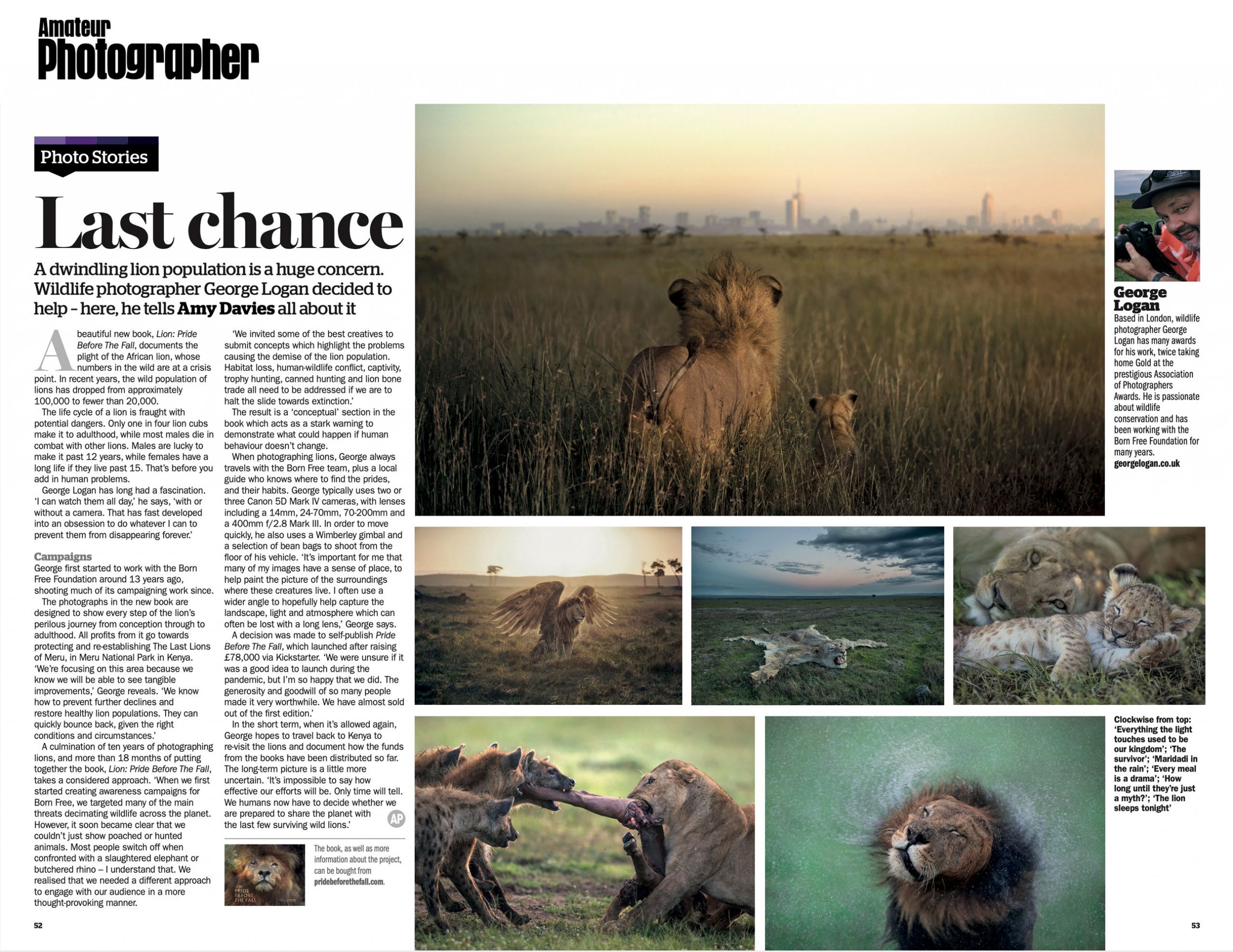In this image, we see an article accompanied by various photographs. The article is presented on a white background with black text. At the top left of the page, it credits Amit Shah as the photographer. Below this, it is labeled "Photo Stories," and the headline reads, "Last Chance: A Twin Leading Lion Population is a Huge Concern. Wildlife Photographer George Logan Decides to Help. Here He Tells Amit Davies All About It."

The article introduces a new book titled "Lion Pride Before the Fall," which beautifully documents the plight of the African lion. It highlights the alarming decline in the wild lion population, which has plummeted from approximately 100,000 to fewer than 20,000 in recent years. 

The first photograph shows a lion and a cub, both with brown fur, standing on green grass and facing away from the camera. In the background, there is a seat and some buildings. On the right side of the page, another image features George Logan, identified as a London-based wildlife photographer with numerous awards, including two golds from the prestigious Association of Photographers Awards. Logan is noted for his passion for wildlife conservation and his longstanding collaboration with the Born Free Foundation (georgelogan.co.uk).

The article includes six additional photographs with detailed captions:
1. A lion with wings.
2. A lion skin laid flat on the ground, with the head still intact.
3. A lion with a lion cub.
4. A dramatic image of a lion and hyenas fighting over a piece of meat; the hyenas are on the left side, and the lion on the right side.
5. A lion shaking its head, splashing water everywhere.

The captions for these photos are listed as follows: 
- "Clockwise from the top, everything the light touches used to be our kingdom."
- "The survivor."
- "Mary Dirty."
- "In the rain."
- "Every meal is a drama."
- "How long until they are just the meat."
- "The lion sleeps tonight." 

This article vividly captures the urgency of lion conservation through compelling imagery and the storytelling of renowned wildlife photographer George Logan.